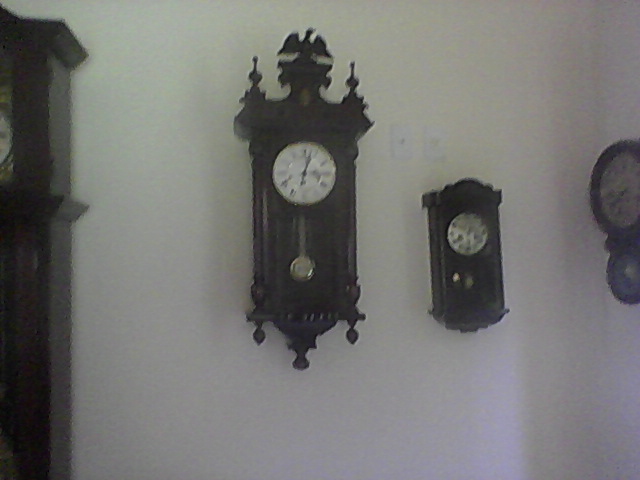The image depicts a portion of an interior wall displaying four antique clocks against a white backdrop. On the far left, partially out of frame, is the side of a tall grandfather clock made of dark wood with a white face. Next to it in the middle, there is an ornate wall-hanging clock with carved posts at the top and bottom, featuring a perched bird, possibly an eagle, at the top. This clock has a white face with black Roman numerals and a gold pendulum encased in the lower part. To its right hangs a smaller rectangular clock, carved from similar dark wood, with a silver face. Finally, the far right showcases another round clock, which also has an off-white face and appears to be in matching brown color as the others. The image has some blurriness, making fine details and the exact time on each clock indistinguishable. Additionally, there are some white wall switches visible, but no text is present in the image.